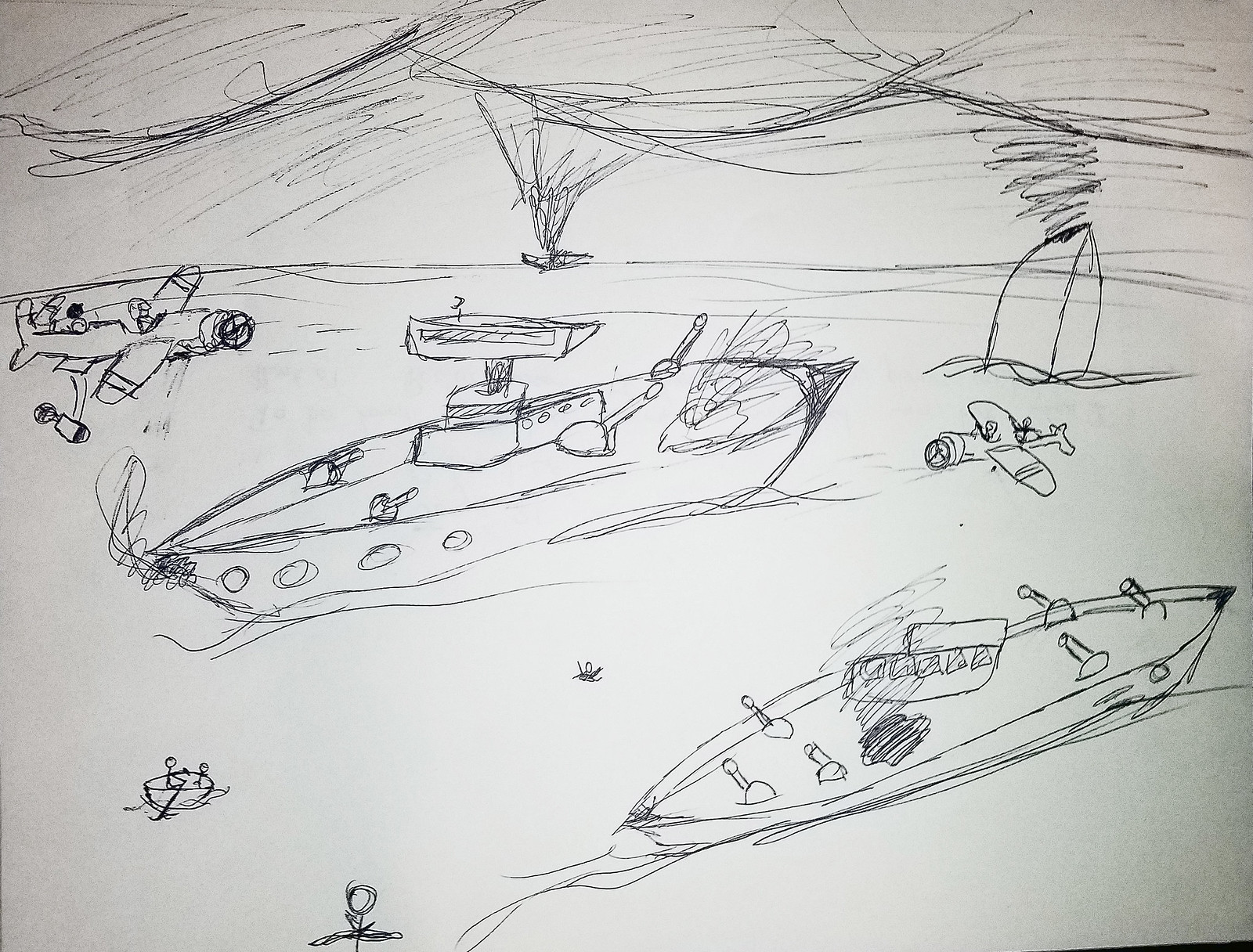A child's hand-drawn picture vividly depicts a wartime scene with remarkable detail. The chaotic background showcases a smoky sky filled with explosions from dropping bombs. In the water, there are multiple ships and airplanes engaged in battle. On the horizon, a small ship appears to be exploding while closer to the left, another ship is seen sinking, with smoke rising from its hull. The scene includes two World War I-era biplanes, one on the right that is actively dropping a bomb. Two battleships with cannons facing each other dominate the sea, with a smaller single-engine plane flying between them. Between these battleships, a person who has fallen into the water is desperately waving for help, with a rowboat approaching to rescue him. Additionally, another person with raised arms is seen closer to the right-hand corner, also awaiting rescue. The intricacies of the drawing reveal visible pilots in the planes and the detailed weaponry, including one ship with six guns on its deck and another with four. The overall composition, although rudimentary in style, is filled with action and conveys the brutal reality of a water and air battle.